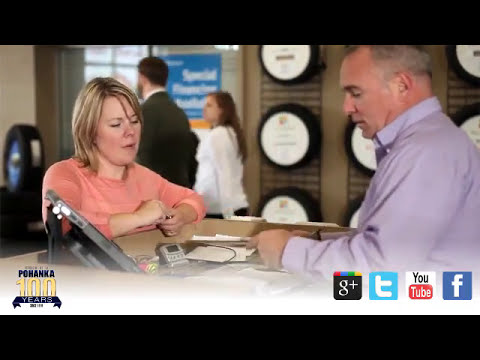The photograph captures an indoor scene centered around a female customer and a retail salesperson engaged at a counter. The woman, approximately 40 years old with shoulder-length blonde hair, is wearing a long-sleeved peach top. She stands with her arms crossed, looking down at some papers on the counter, facing the salesperson. The salesperson, a man around 50 years old with thin salt-and-pepper hair, is dressed in a long-sleeved lavender shirt and is also focused on the counter. Situated in the lower left-hand corner of the image, there is a logo reading "Pohakana, 100 years" in tall gold lettering, accompanied by links to social media platforms like Google+, Twitter, YouTube, and Facebook in the bottom right corner. The background is slightly blurred, revealing award plaques with white circles on a wall and two additional customers—a man in a black top and a woman in a long-sleeved white top—moving around. The overall style of the photograph is one of photographic representationalism, resembling a freeze-frame from a video.